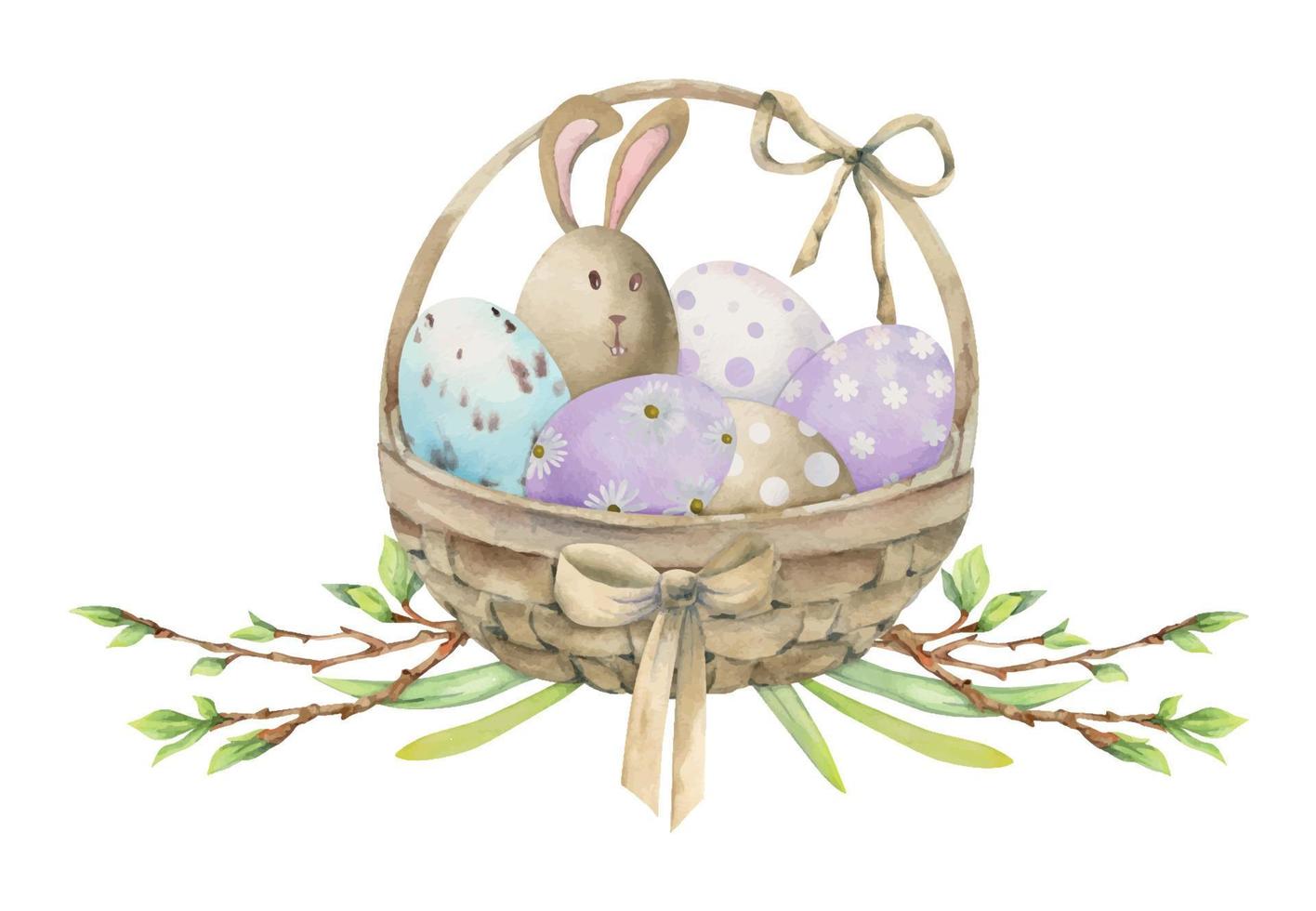This computer-generated image against a solid white background showcases a light brown wicker basket accented with bows. One bow is tied in the front, and another adorns the handle on the upper right side. The basket contains approximately six artistically decorated eggs, each with unique designs and hues: one is solid brown with a bunny face, complete with ears, eyes, a nose, and teeth; another is blue and white with brown spots; and there are two purple eggs—one features flowers with white petals, while the other boasts white petaled flowers. Additionally, there is a white egg with purple polka dots and a brown egg with white polka dots. Emerging symmetrically from either side of the basket are brown twigs and branches adorned with green leaves, adding a touch of natural elegance to this Easter-themed artwork.